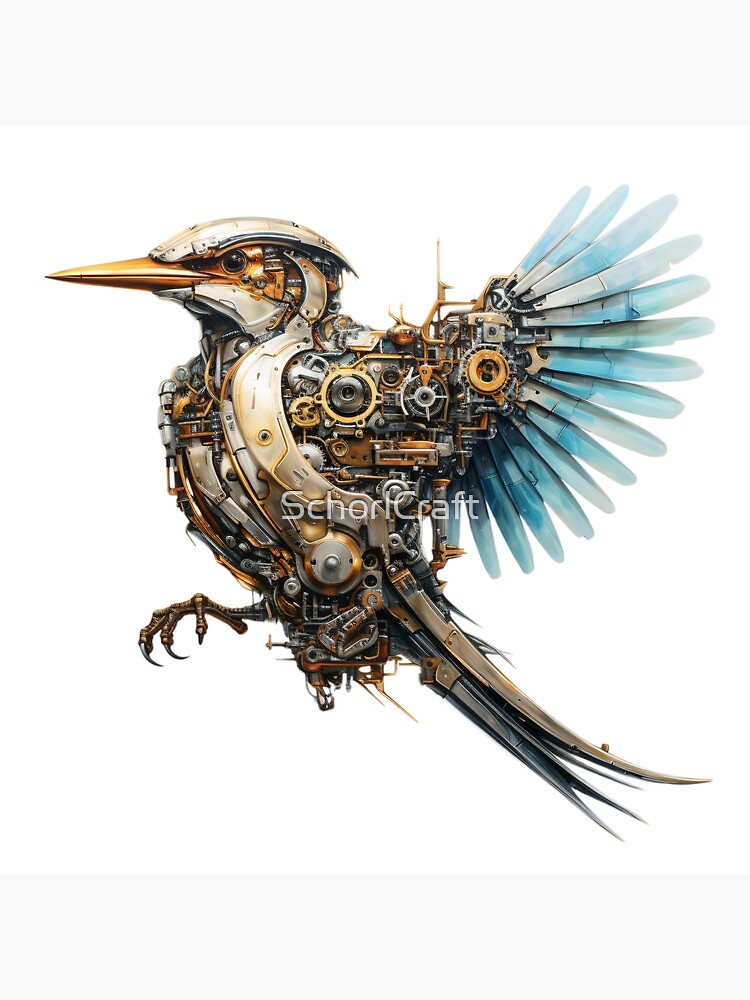This image is a highly detailed drawing of a robot bird facing left, offering a side view of its intricate design. The bird features metallic elements with a shiny finish, giving it a futuristic and mechanical appearance. Its long beak is a goldish brown color, while the head is a light brown, and the dark-colored eyes provide a stark contrast. The body of the bird is primarily silver, exposing a complex array of gears, wires, pipes, and other mechanical parts. It resembles the inner workings of a skeletonized watch, with various metallic colors such as shiny silver steel, copper, and brass.

The wings are designed with blue, fan-like feathers that have the appearance of metal fans, and the tail also incorporates elements of blue and silver. The bird’s talons are made of brass-colored metal with sharp black claws. This mixture of materials and mechanical components makes it look like an unfinished robot with its outer plating removed, revealing a fascinating interior.

Additionally, the image has white text in the middle that reads "SCHORLcraft," and it is set against a white background with gray bars at the top and bottom of the image, further emphasizing the bird's mechanical features.